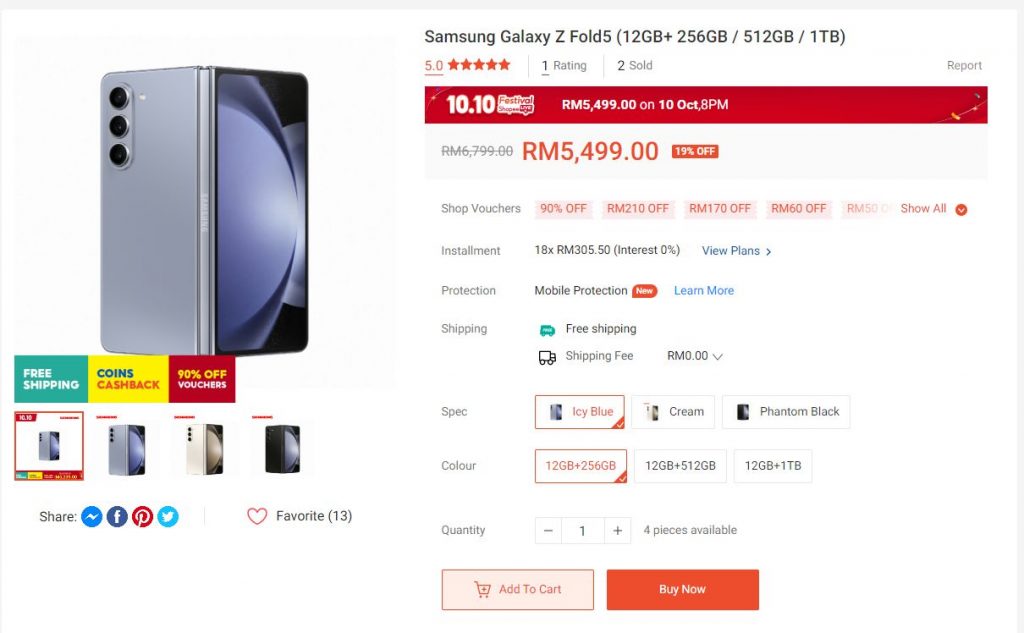This screenshot from an unidentified shopping website features a detailed listing for the Samsung Galaxy Z Fold 5. On the left side, there's a prominent photograph of the foldable cell phone, capturing both the screen and the back. The phone is displayed in its folded state, revealing a sleek gray back with three vertically aligned camera lenses and a dynamic wallpaper on the screen featuring a blue shape against a black background. 

Various angles of the phone are shown, including models with a steel gray back, a white back, and a black back. The listing header includes options such as “share” and “favorite,” with a count of 13 favorites.

To the right, the product is identified as the "Samsung Galaxy Z Fold 5" with options for 12GB of RAM and three storage capacities: 256GB, 512GB, and 1TB. It has a five-star rating from one review, and only two units have been sold. There's a mention of a festival event on October 10 with a specific price listed, RM 6799.00, which has been crossed out and replaced with a discounted price of RM 5,499.00 (19% off).

The listing elaborates on available discounts and vouchers, including offers like 90% off, RM 210 off, RM 170 off, and RM 60 off. Additionally, there are installment options (18 installments of RM 305.50 at 0% interest) and mobile protection plans.

Shipping is free (fee: RM 0.00). The spec options include colors like icy blue, cream, and phantom black, with icy blue selected. Storage options available are 12GB RAM with 256GB, 512GB, or 1TB storage, with the 12GB/256GB combination highlighted. The stock indicates four pieces available, with buttons to add to the cart or buy immediately.